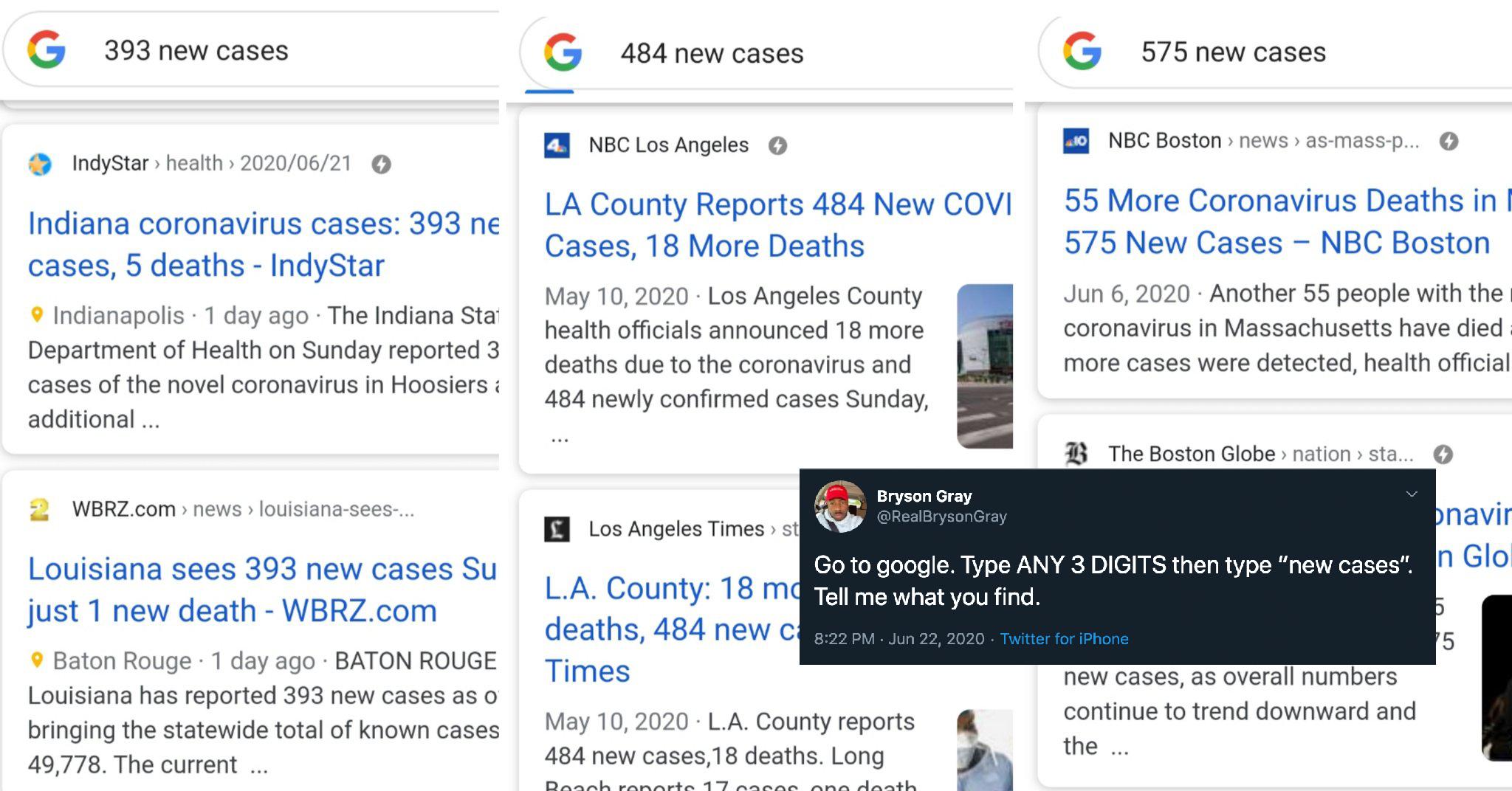Here's a detailed and cleaned-up caption for the image:

---

The image depicts a web page, resembling a Google search results screen, displaying various news snippets about COVID-19 cases. The layout is divided into three columns.

**First Column:**
- At the top, there is the familiar Google logo alongside a summary: "393 new cases."
- Directly below, two articles are listed:
  - The first article is from "IndyStar Health" dated June 21, 2020. The headline reads: "Indiana coronavirus cases: 393 new cases, 5 deaths - IndyStar."
  - The second article is by "WBRZ.com News" and reports: "Louisiana sees 393 new cases, just 1 death - WBRZ.com."

**Middle Column:**
- The top features a prominent Google search bar.
- Below the search bar, the content includes:
  - "484 new cases" reported by "NBC Los Angeles News." The headline states: "LA County reports 484 new COVID cases, 18 more deaths."
  - Another article from the "Los Angeles Times" is partially covered by a Twitter post from Bryson Gray, reading: "Go to Google, type any three digits, then type 'new cases.' Tell me what you find."

**Third Column:**
- At the top is a Google search summary: "575 new cases."
- The primary news snippet is from "NBC Boston News" with the headline: "55 more coronavirus deaths and 575 new cases - NBC Boston."

Overall, the image presents a snapshot of how different news outlets report on COVID-19 cases, organized neatly in a grid resembling a Google search results page.